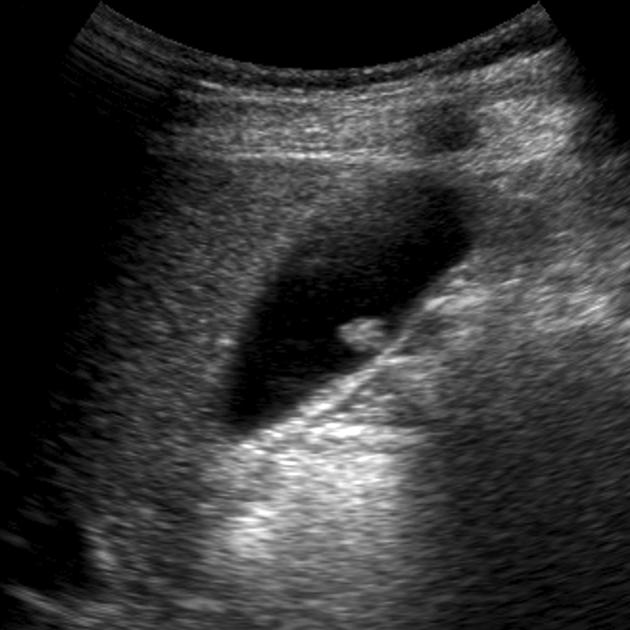This image appears to depict an ultrasound scan with a predominantly black background and various shades of gray forming the central focus. The grayscale coloration and the distinct variation between black, white, and gray patches strongly resemble the visual characteristics typical of ultrasound imagery. The image itself is vertically oriented and shaped somewhere between a square and a rectangle. Within the scan, there is a prominently defined black area that likely represents an empty part of the uterus, bordered by the gray contours that outline the internal view of the body. Inside this black region, early signs of a developing fetus are discernible, manifesting as a small, oblong cluster that may indicate the initial stages of pregnancy. While there are no labels present to provide additional context, the clarity and structure of the image suggest a well-taken ultrasound, giving a glimpse into an early pregnancy state.